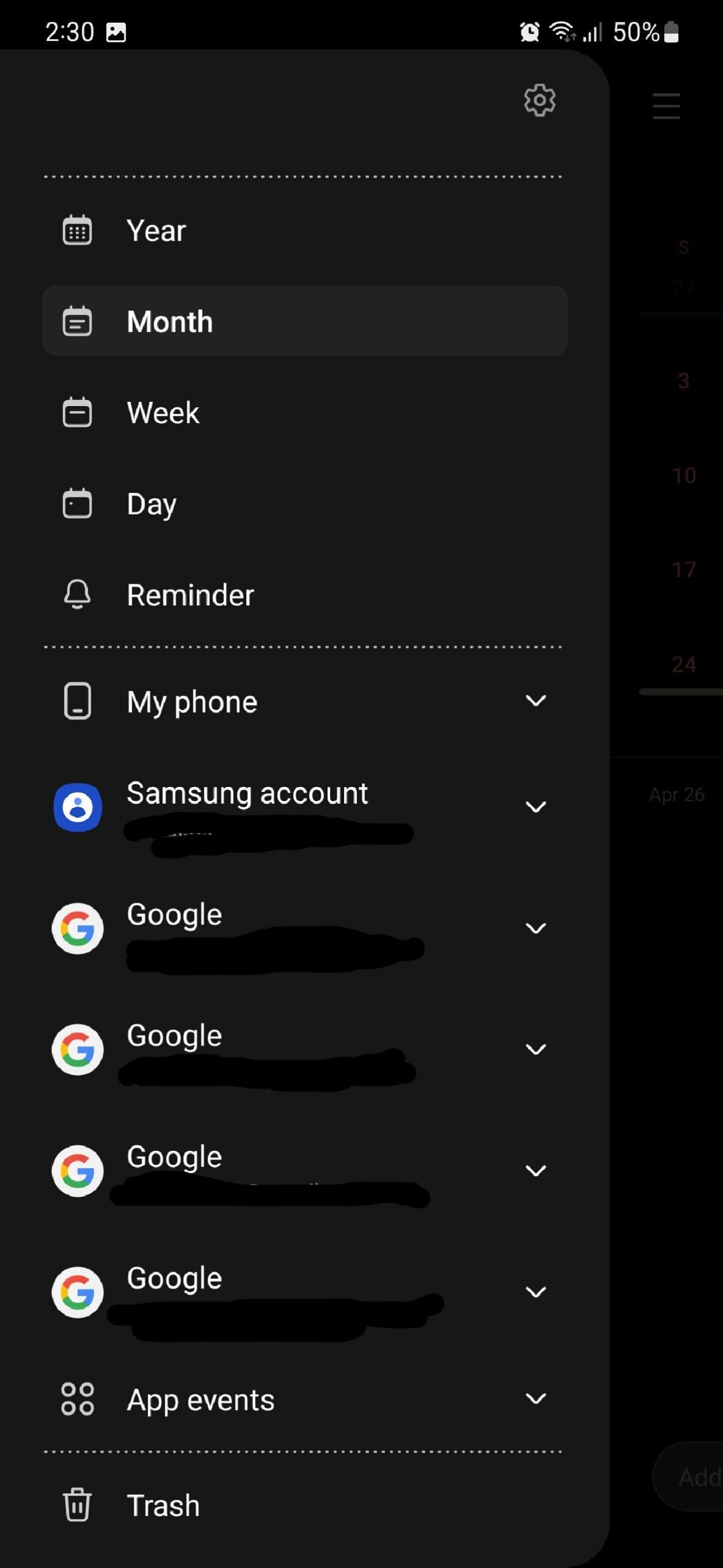The image displays a smartphone screen with various interface elements and settings. In the top left corner, the time "2:30" is visible. On the right side of the screen, icons illustrate the status of different functionalities, including an alarm clock, Wi-Fi connectivity, signal strength, and a battery indicator showing 50% remaining. Beneath these icons, a cogwheel symbol representing the settings menu is present.

Along the left-hand side of the screen, a series of titles accompanied by corresponding icons is listed. These titles include "Year," "Month," "Week," "Day," and "Reminder." Below this section, another category showcases account-related options such as "My Phone," "Samsung Account," and multiple entries labeled "Google." Notably, the four Google entries and the Samsung account have details obscured by black scribbles to protect the user's personal information. Each item in this section features a pull-down menu that allows users to expand and access specific settings.

At the bottom of the screen, there is a section labeled "Trash." The far right side of the screen is depicted as a plain black panel, providing a visual contrast to the detailed left side.